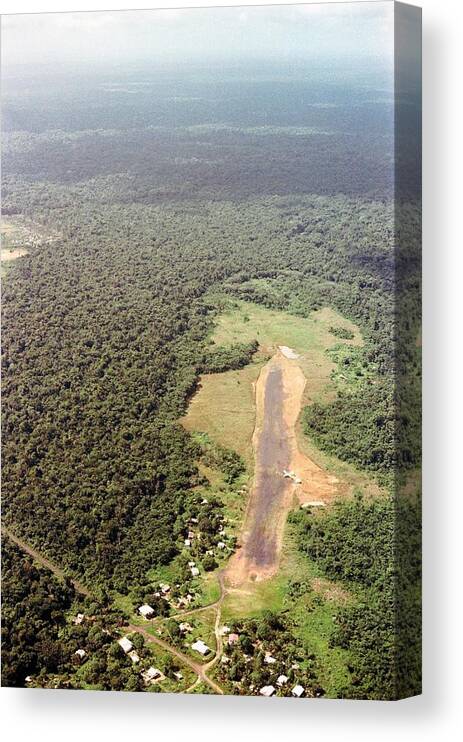This detailed canvas print captures an aerial view of a verdant landscape, likely in a region such as Columbia. The scene depicted is surrounded by a white background and is set on a slightly tilted vertical rectangle, giving it a three-dimensional appearance as it wraps around the sides of the canvas. The upper portion of the image shows a sliver of blue sky with scattered clouds.

In the middle of the print, you can see a small village composed of white buildings nestled amidst a grassy area. A prominent dirt trail leads into the village, flanked by dense clusters of dark green trees that extend to the horizon, becoming even darker green with distance. A significant feature of the composition is a vertical rectangular strip of brown dirt slightly to the right of center, which seems to cut through the greenery, possibly indicating a landing strip or a similar cleared area. Surrounding the village and the dirt strip are various dirt roads and scattered housing developments, all of which contribute to the impression of a remote, expansive rural community captured from above.